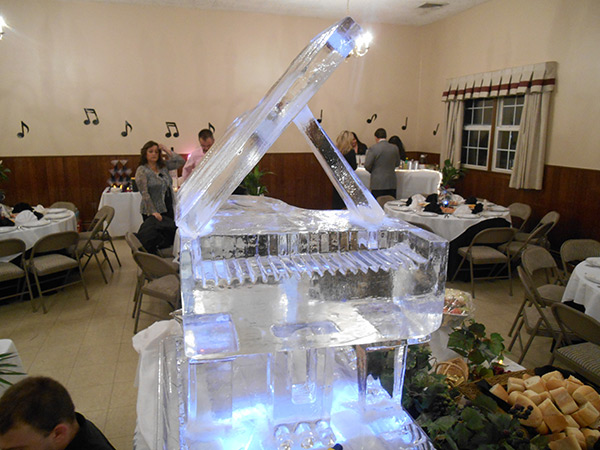The image depicts a party or function set in a large room. The room features a tile floor with underlying wood, whitewashed walls, and wooden wainscoting. There are some windows with curtains, described as quite plain. In the background, musical notes are displayed on the white walls, perhaps hinting at a musical theme or celebration. Round tables with folding chairs are arranged around the room, all set with plates and possibly drinks, indicating that the event involves dining.

At the center, a prominent table stands out with an assortment of bread, buns, and croissants, suggesting it is a focal point for refreshments. The main highlight of the image is an intricately carved grand piano ice sculpture sitting on this table. The sculpture is impressive, with details such as the lifted top, keys, and pedals all carefully crafted from ice. Illuminated to draw attention, this ice piano acts as the centerpiece of the room.

Attendees are mingling around the room, mostly standing rather than sitting, giving the impression that the event is still in its early stages. The overall ambiance suggested by the severe wooden wainscoting and plain fixtures contributes to a somewhat austere, possibly post-communist Eastern Bloc aesthetic.